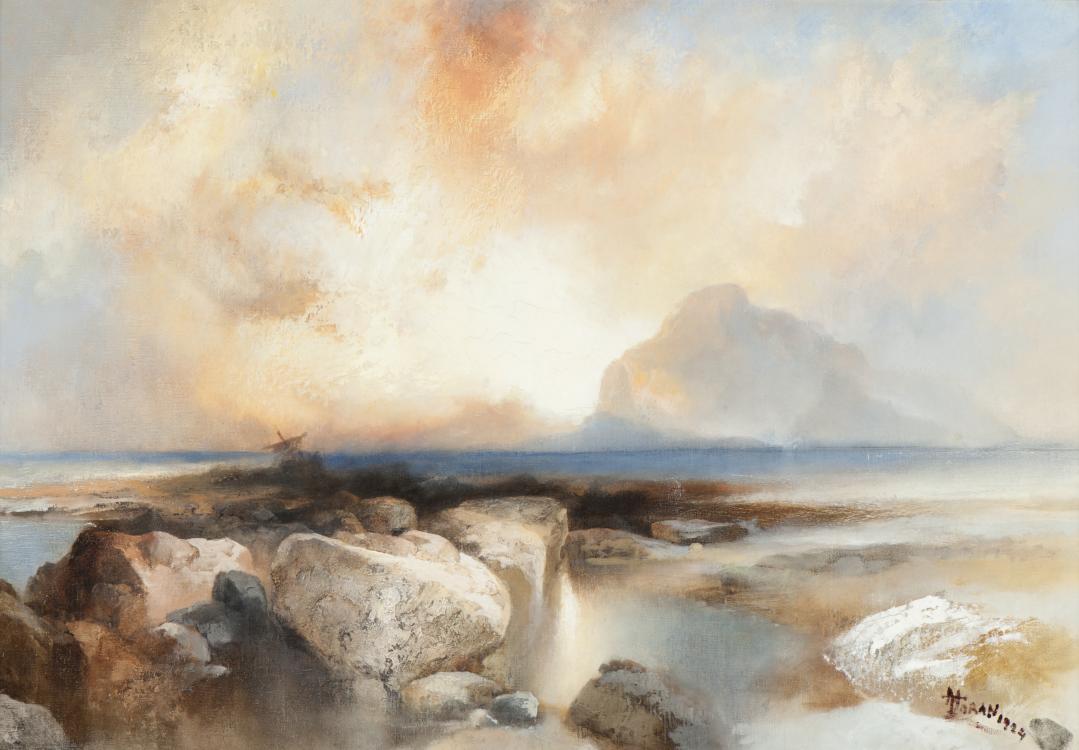This painting, titled "Seascape," presents a dramatic and evocative seashore scene. The top half of the image displays an apocalyptic sky with a bright sun piercing through white and pale orange clouds, creating a surreal mix of colors reminiscent of a sunset. The lower half features an empty beach scene with large, white rocks in the foreground, some showing signs of water spilling over them, forming small tidal pools. The beach extends to the horizon on the right, with brown sand and traces of dirt. To the left of the frame, there's a shoreline inlet with ocean water lapping against the rocks. In the background, a shipwreck with a visible sail seems stranded on the coast, emphasizing the desolate atmosphere. The overall style of the painting has a slightly washed-out effect, possibly due to the intense sunlight, enhancing the deserted and eerie nature of the scene.